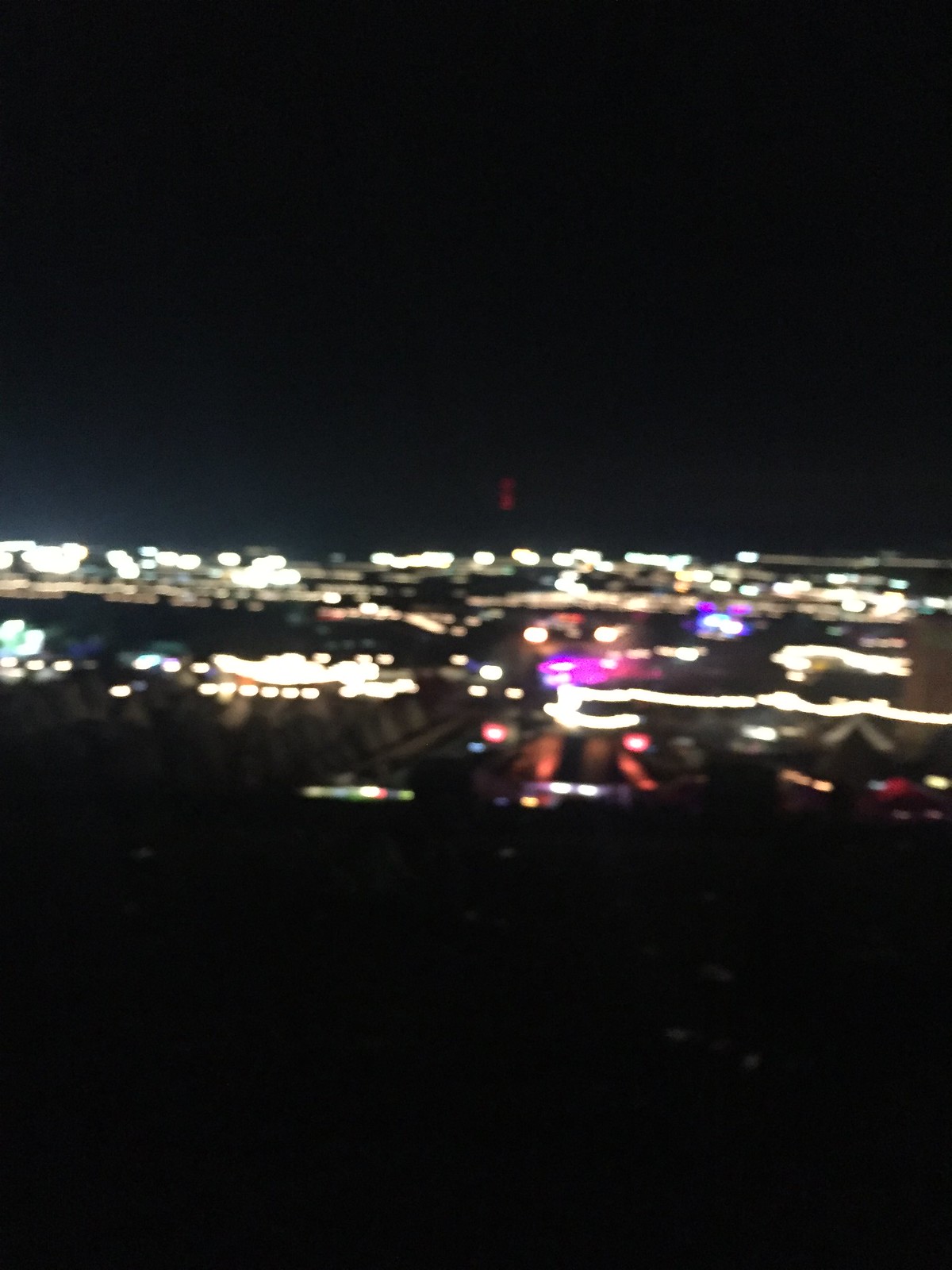The photo presents a blurry, nighttime city skyline, likely of Las Vegas, taken from a distance. The image is dominated by a dark background with the top and bottom largely obscured in blackness. The central area of the photo is illuminated with myriad lights of various shapes and colors. Predominantly white lights intermingle with hues of purple, blue, pink, and orange. Some lights appear as small, round dots while others are longer and more linear. A bridge might be discernible in the center, flanked by diverse light patterns. Among the colorful lights, areas of the center-right display blue, circular lights, which could suggest emergency vehicles. Faint, indistinguishable objects and whitish circles are visible toward the bottom right, adding to the complex yet vibrant atmosphere of the cityscape.